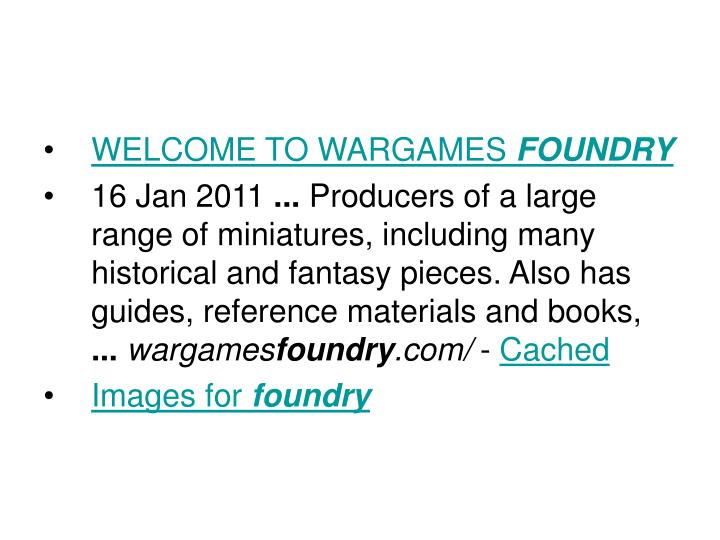The image depicts a PowerPoint slide with a white background, featuring three bullet points. The first bullet point reads, "WELCOME TO WARGAMES FOUNDRY," written entirely in teal, Arial font, and underlined. The word "FOUNDRY" is both bolded and italicized. The second bullet point lists the date "16 Jan 2011" followed by descriptive text: "Producers of a large range of miniatures, including many historical and fantasy pieces. Also has guides, reference materials, and books." The URL "wargamesfoundry.com" is included, with the word "cached" in teal, underlined, indicating a hyperlink. The third bullet point says "Images for Foundry," also in teal, underlined, and with "Foundry" bolded and italicized.